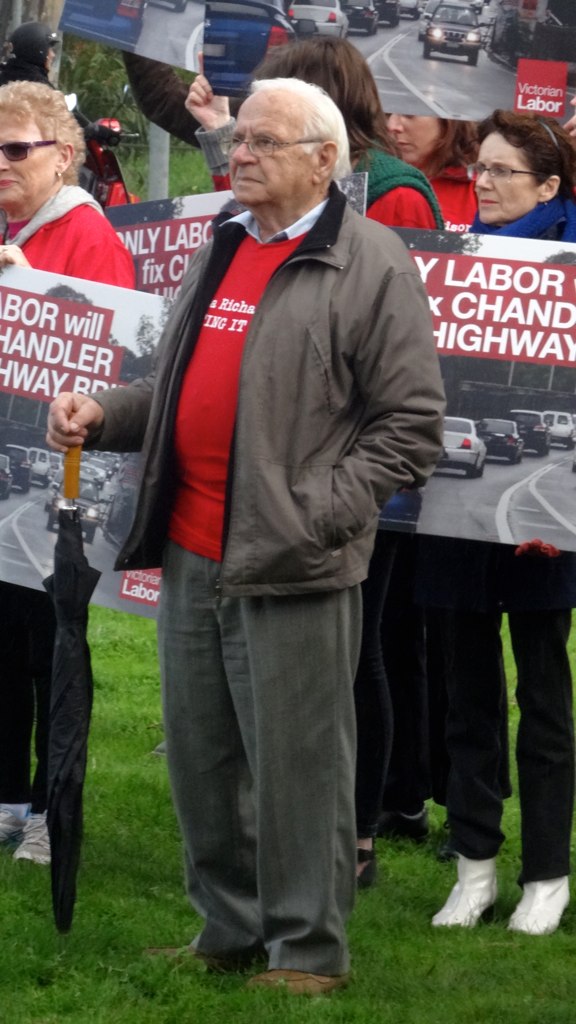The image depicts a crowd of people gathered outdoors, seemingly on a grassy area, taking part in a protest rally. Prominently in the foreground stands an elderly man, possibly in his 70s, with gray hair and glasses. He is dressed in a red sweater layered over a collared shirt, paired with gray slacks and a gray jacket, and is holding an umbrella. Surrounding him are other individuals holding signs with partial messages visible, including the words "labor" and "highway," alongside traffic imagery. Most of the participants are wearing red shirts, suggesting a coordinated effort. Although the specific details of the protest are unclear, it appears to be related to labor issues, possibly advocating for labor workers in relation to highway construction. In the background, you can also spot a road with cars passing by, adding to the context of the gathering.